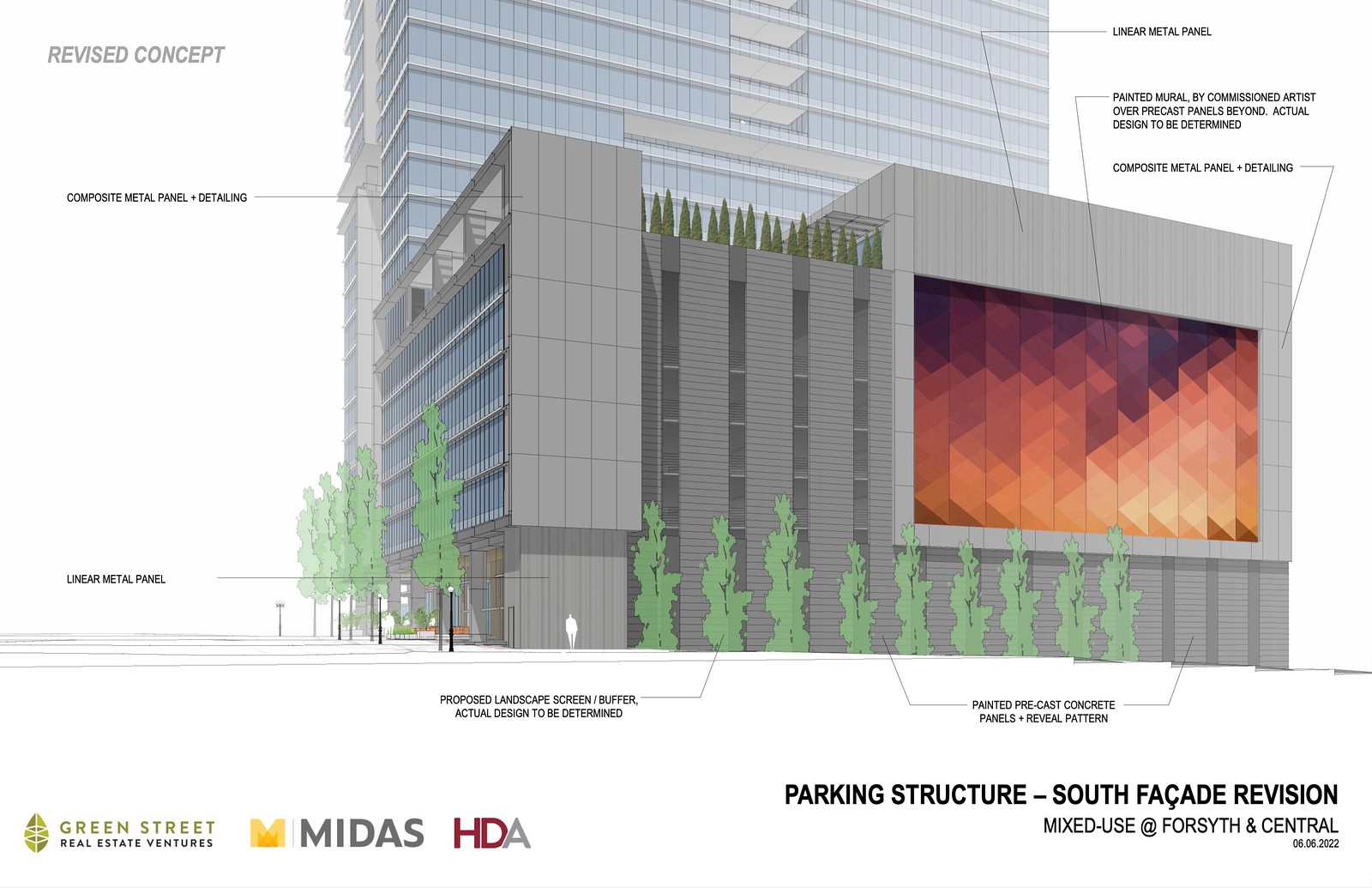This is a detailed architectural drawing, rendered using computer software, of the south facade revision of a planned multi-story parking structure adjacent to a larger building, dated June 6, 2022, and located at Forsyth and Central. The facade is depicted in a stylized, almost cartoony manner. The building features gray siding with numerous windows. A significant visual element is the large painted mural, featuring orange, dark purple, dark blue, and various light orange hues, by a commissioned artist over precast panels, with details yet to be finalized.

The image is annotated with several labels pointing to specific architectural elements: "linear metal panel," "composite metal panel plus detailing," and "painted precast concrete panels and reveal pattern." Additionally, the proposed landscape screen/buffer with trees is indicated along the walkway surrounding the building. The design is marked as a revised concept in the top left corner.

The bottom of the image includes logos and text for Green Street Real Estate Ventures, Midas, and HDA, and the bottom right corner is labeled with "Parking Structure, South Facade Revision" along with the project details.